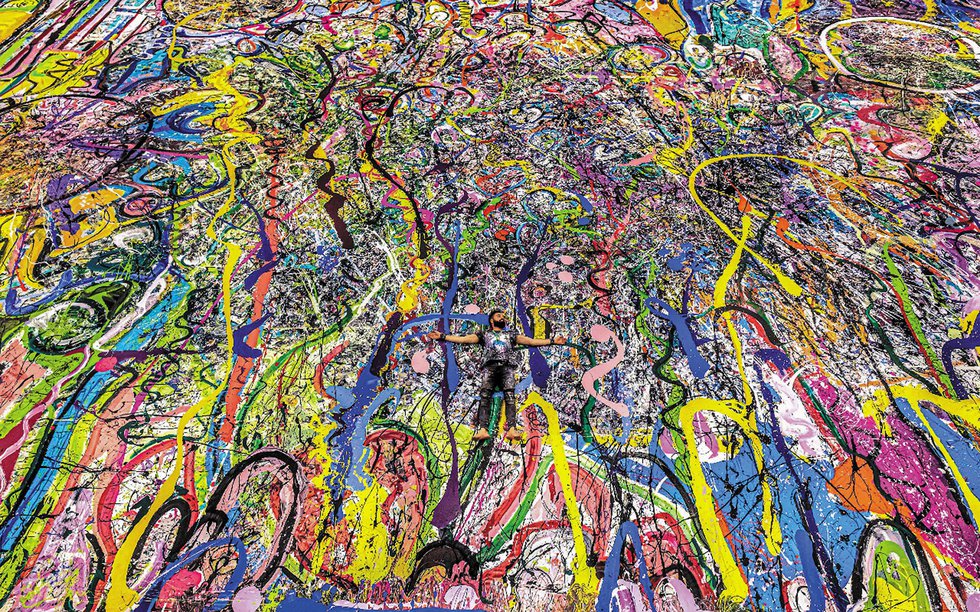The painting in question is a vibrant, abstract expressionist work reminiscent of Jackson Pollock, characterized by a flurry of swirling colors and dynamic lines in shades of yellow, red, blue, black, and more. The canvas is densely packed with chaotic, yet somewhat orderly brushstrokes that seem to be thrown onto the surface, creating a sense of energetic movement. Amidst this colorful turbulence, just below the midway point, there is a small, distinct depiction of a male figure. This figure, with black beard and hair, is painted with outstretched arms, seemingly in a pose of celebration or exultation. Details such as black wristbands, a short-sleeved top, dark pants, and possibly white boots and bare legs can be discerned. The figure appears to be light-skinned and is surrounded by a burst of colorful lines and shapes that dominate the canvas, creating a sense of being enveloped in the artist’s frenetic and passionate creative process.